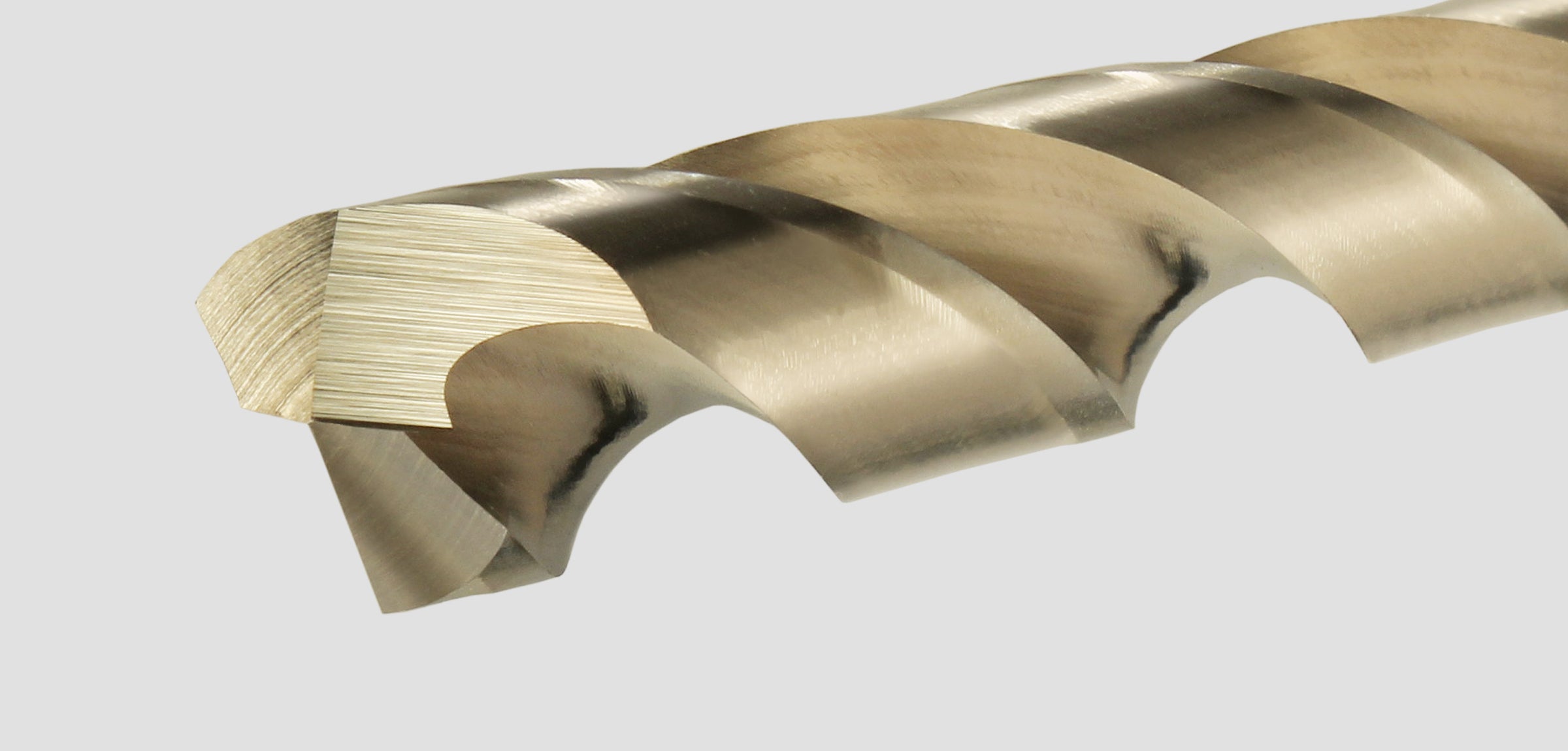The image is a detailed close-up of a golden metal drill bit, occupying approximately half of the frame. The drill bit enters the image diagonally from the upper right corner, extending downward towards the lower left. It showcases intricate details, including the coiled spiral pattern that is characteristic of drill bits, with raised and sunken areas adding to its textured appearance. The surface of the bit is polished, with visible striations and grain marks that highlight the craftsmanship. The tip of the drill bit, which comes to a slight point, is positioned towards the lower left side of the image. The drill bit's coloration varies from black and gray to brown and light beige, indicating a shiny reflective surface, likely due to a light source coming from the right. Three distinct facets at the very end of the bit reveal variations in color and texture, with one looking gray and others appearing brown. The background is a very light gray, providing a neutral backdrop that contrasts with the striking metallic hues of the drill bit.